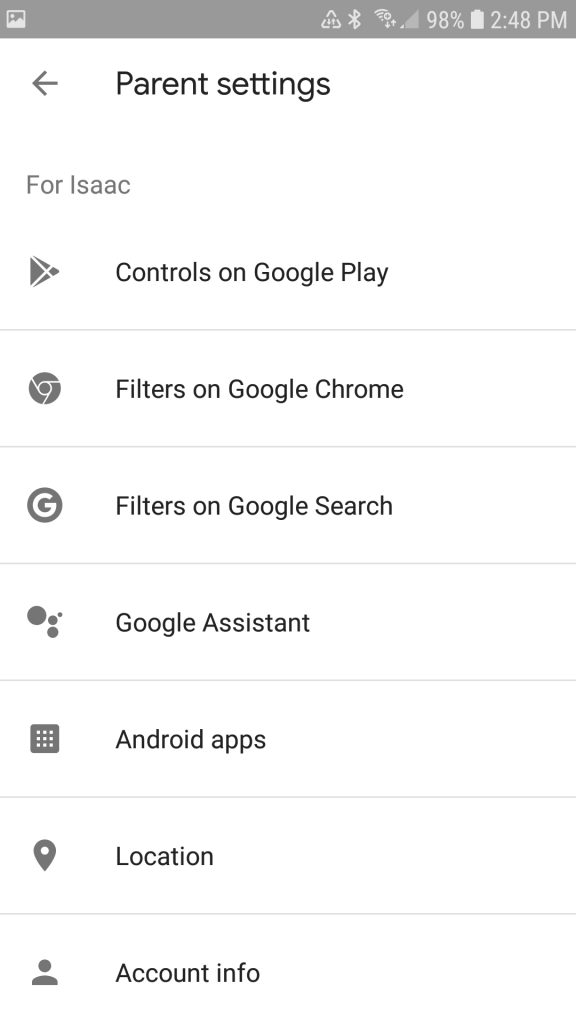The image displays the Parental Settings interface for Google, clearly tailored for a user named Isaac. At the top of the screen, the title "Parental Settings" is prominently displayed in bold letters. Just beneath this, it indicates the settings are specifically for Isaac. The interface details various control options, each accompanied by relevant icons. These options include:

- **Controls on Google Play:** Marked by the Google Play Store icon.
- **Filters on Google Chrome:** Accompanied by the Google Chrome logo.
- **Filters on Google Search:** Identified by a black circle with a white "G."
- **Google Assistant:** Represented by four colored circles.
- **Android Apps:** Denoted by a square containing white circles.
- **Location:** Illustrated with a pin icon.
- **Account Info:** Symbolized by a little person icon.

Additionally, there is a back arrow at the top left corner, indicating navigation options to other parts of the device. 

At the top of the screen, the device status shows a 98% battery charge and the current time as 2:48 PM.